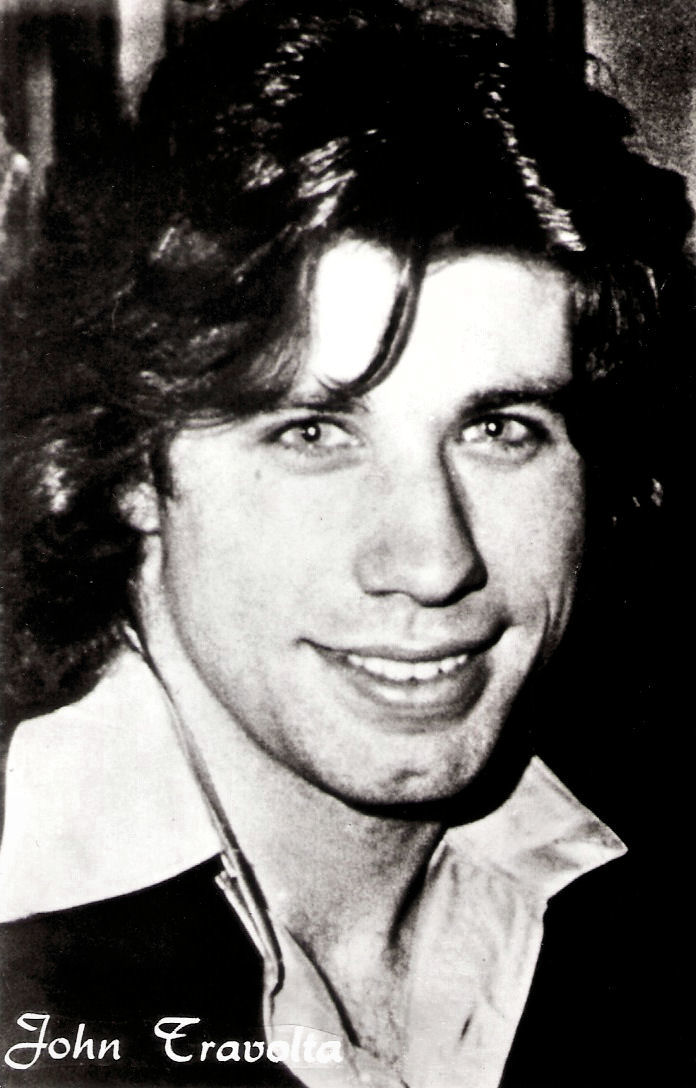This image is a vintage black-and-white promotional photograph of John Travolta, likely from the 1970s, possibly tied to his roles in "Welcome Back, Kotter" or "Saturday Night Fever." The head-and-shoulders close-up captures him smiling directly into the camera, with his teeth visible and a youthful exuberance. Pictured in a 1970s-style shirt with a wide collar open at the neck, hints of chest hair peek through the V-neck. His hair is long and slightly greasy, with a strand falling over his right eye (to the viewer's left) and extending down to his shoulders. The photograph includes a white cursive watermark on the bottom left corner reading "John Travolta." The image, taller than it is wide, features no visible background, focusing entirely on Travolta's face and upper torso.